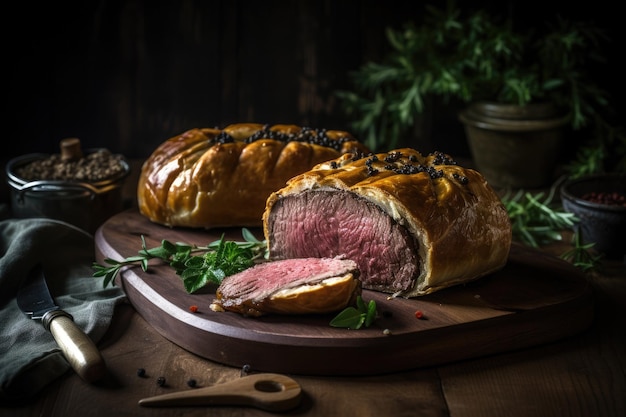The image depicts a piece of Beef Wellington, a dish featuring rare beef wrapped in a golden-brown crust. The meat, sliced open to reveal its pink and tender center, rests on a dark wooden cutting board alongside a knife with a wooden handle. Surrounding the Beef Wellington is a garnish of fresh parsley, adding a vibrant touch. Scattered small black berries or seeds adorn the dish, enhancing its visual appeal. In the background, another uncut Wellington sits alongside a pot and vases with green plants, adding a touch of natural decor. The overall presentation is richly detailed, with elements like a bowl and wooden utensils subtly visible, creating a warm and rustic culinary scene.